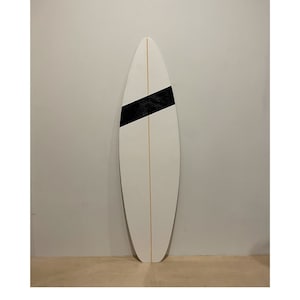The image showcases a surfboard prominently positioned in the center, standing upright and leaning against a white wall with light tan wood flooring beneath. The surfboard, which is predominantly white, features a distinct tan stripe running vertically down its middle. Additionally, there is a bold, diagonal black stripe that cuts across the upper half of the board, slanting from right to left and starting higher on the right side. The surfboard has an oval shape with a pointed top and a broader base resting on the floor. The scene appears to be indoors, likely within a home, given the clean white wall and light-colored flooring, and there are no people or text present in the image.